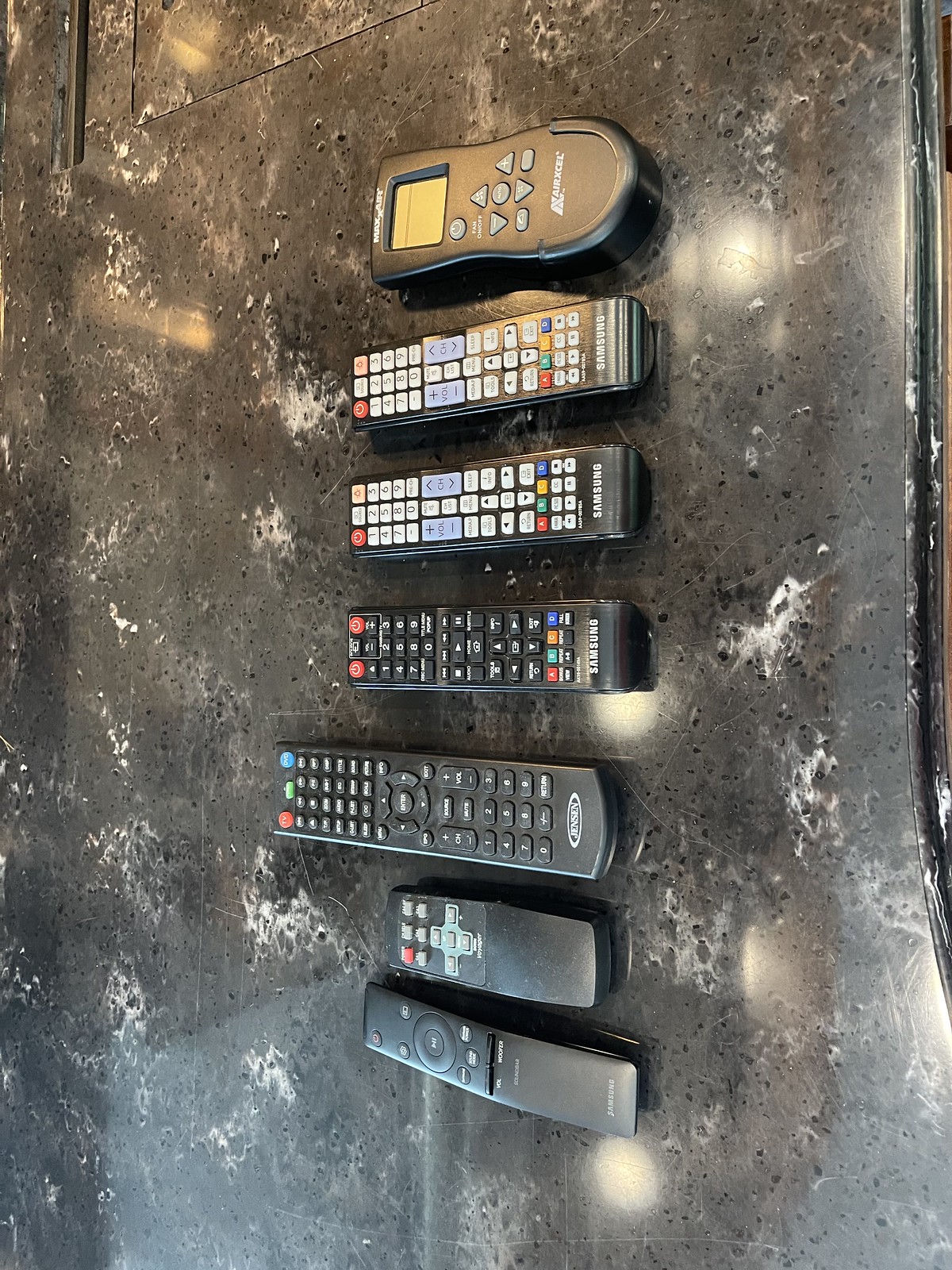A photo depicts a vertical arrangement of seven remote controls placed on a dark gray granite countertop with white splashes. The remotes, which vary in design and button complexity, are primarily black with multi-colored buttons and white text. Starting from the bottom, the first three remotes showcase different layouts: a thin remote with few buttons, a slightly thicker remote with a central dial, and another basic remote with minimal buttons. The next three remotes are all labeled Samsung and resemble universal remotes, each jam-packed with buttons. The final remote appears unique and more intriguing, having a peanut shape with an LCD screen on top, resembling a high-tech garage door opener rather than a TV remote. The image, taken from an angled, side-on perspective, requires tilting one's head sideways to read any labels. Overall, the remotes lay parallel to each other, prominently highlighting their diverse designs against the distinctive marbled countertop.